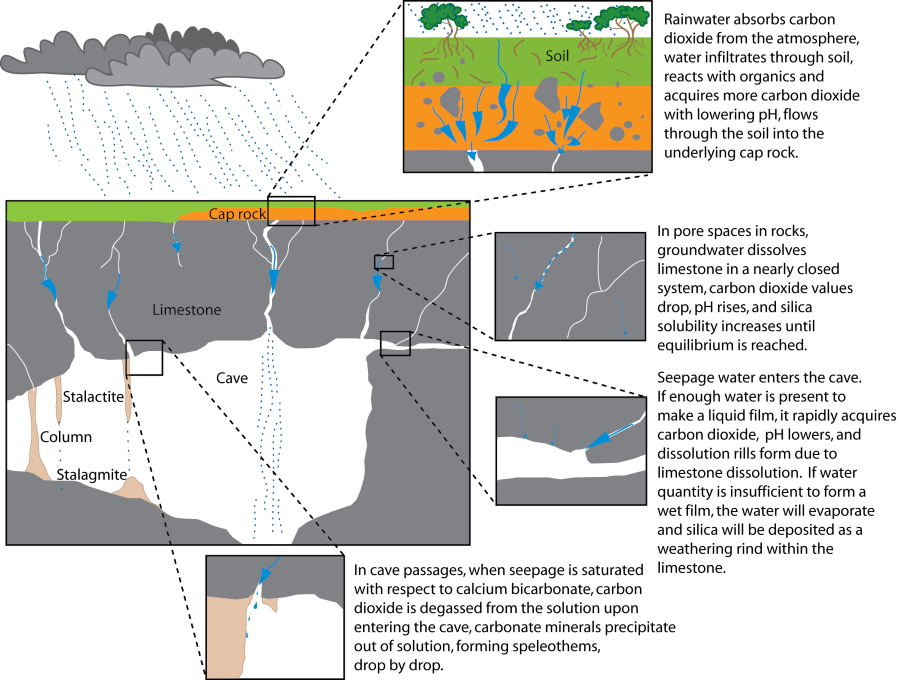This detailed textbook diagram illustrates the process of groundwater infiltration and formation of cave structures such as stalactites and stalagmites. The image shows rainfall absorbing carbon dioxide from the atmosphere before infiltrating through various layers of soil and interacting with organic materials, which further increases CO2 levels and lowers the pH. As water percolates deeper, it passes through the upper, lower, and bottom layers of soil, eventually reaching the underlying cap rock and limestone.

The diagram elaborates on how groundwater moves through pore spaces in the rocks, dissolving limestone in a nearly closed system where CO2 values drop, pH rises, and silica solubility increases until equilibrium is achieved. Seepage water then enters cave systems as long as there is enough moisture to form a liquid film. This film rapidly acquires CO2, lowering its pH and causing limestone dissolution. Alternatively, if water is insufficient to form such a film, it evaporates, leading to the deposition of silica as a weathering rind on the limestone.

On the right side of the main image, there are descriptions and detailed call-outs that explain these processes further. These call-outs specifically highlight how groundwater permeates through different soil layers and enters cave systems. Seepage saturated with respect to calcium bicarbonate degasses CO2 upon entering the cave, causing carbonate minerals to precipitate and form speleothems including stalactites and stalagmites drop by drop. This comprehensive diagram might be found in a geology textbook or educational material describing the water cycle and formation of cave structures.